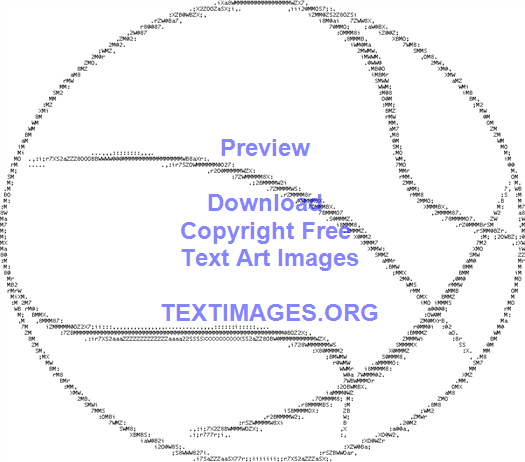The image features a line drawing of a soccer ball with a predominantly white background. The soccer ball, which appears faintly pixelated or fuzzy, is meticulously composed of numerous tiny numbers and letters that create a dizzying effect upon close inspection. Notable numbers, such as "72" and "EX," are barely discernible within the intricate design. Positioned in the center of the soccer ball, in bold purple text, are the words "PREVIEW." Directly below, it continues with "DOWNLOAD COPYRIGHT FREE TEXT ART IMAGES" in smaller purple font, followed by "TEXTIMAGES.ORG" in all caps on the final row.